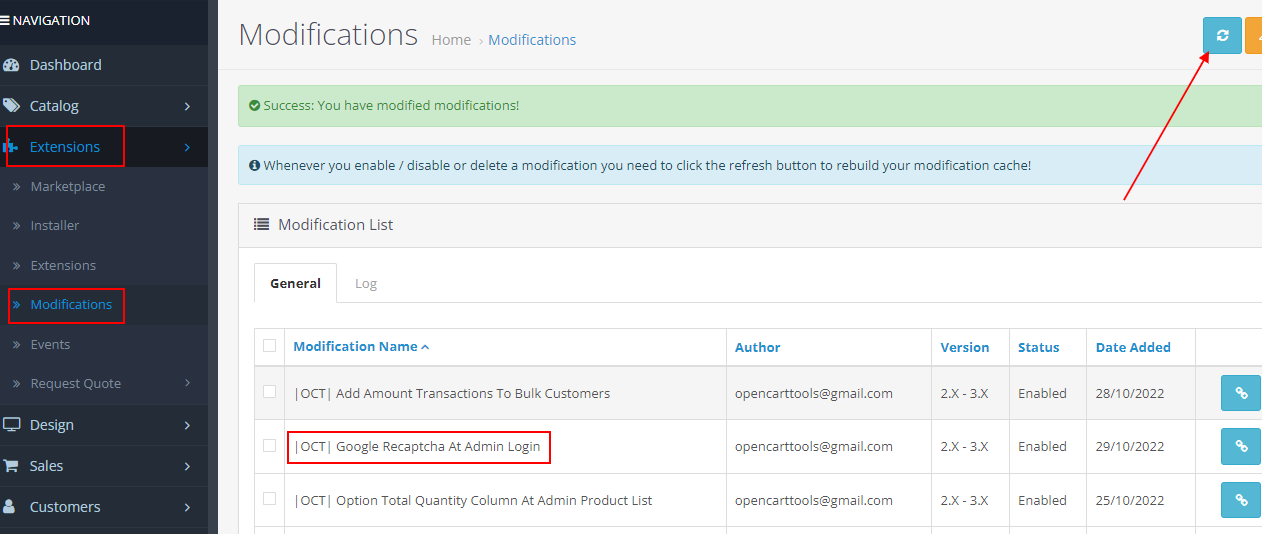![Screenshot of Modification Section in OpenCart Administrative Dashboard]

This detailed screenshot showcases the 'Modification' section within the 'Extensions' area of an administrative dashboard, presumably for a website management tool like OpenCart. The interface is divided into two primary sections: a left-hand navigation panel and a main content area.

On the left-hand side, the navigation panel includes a variety of links for managing different aspects of the website. These include Dashboard, Catalogue, Extensions, Design, Sales, Customers, and others. The Extensions section is expanded, displaying a submenu with 'Modifications' selected.

In the main content area, we see the 'Modifications' page. At the top, a green success message reads, "Success: You have modified modifications!" directly beneath this, an instruction prompts the user to "Click the refresh button to rebuild the modification cache."

This page is divided into two tabs: 'General' and 'Log.' Under these tabs is a list titled 'Modification List' which contains columns for Name, Author, Version, Status, and Date Added.

The first row in this list is 'OCT Google reCAPTCHA at Admin Login' by 'opencarttools@gmail.com,' and its status is 'Enabled,' with the addition date listed as '28/10/2022.' Highlighted with a red arrow pointing towards it is a 'Refresh' button, emphasizing the need to click it to apply recent changes.